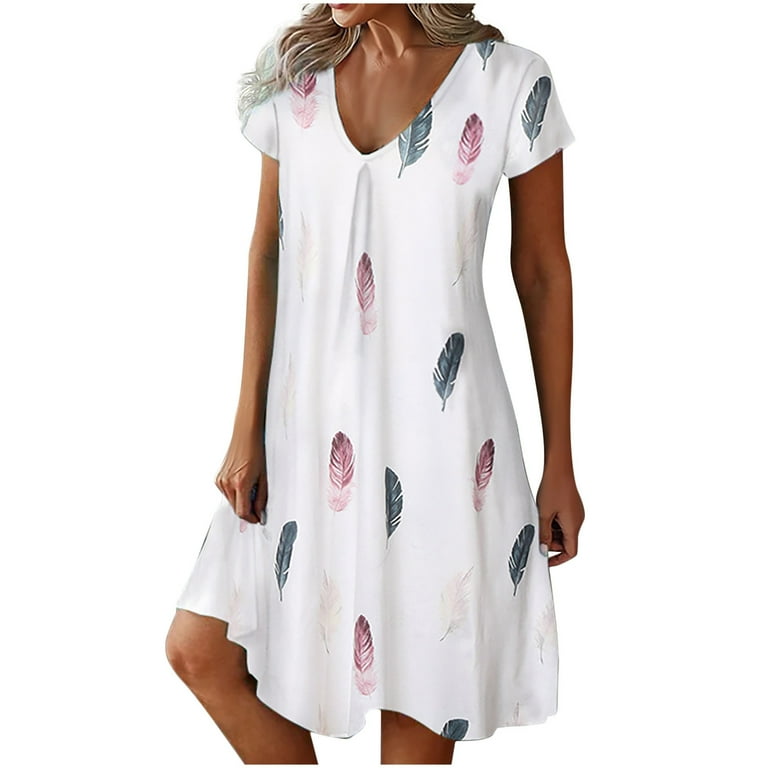The image features a photograph of a model showcasing a semi-tan woman with long, shoulder-length blonde hair wearing a white, summer-like dress adorned with a pattern of pink, green, and faint white feathers. The dress is designed with short sleeves, a V-neck, and a loose, flowy bottom. The photograph captures the model from just below her lips to her calves, with her left knee slightly bent as she poses, holding her hands at her sides. The dress's hemline reaches slightly above her knees in the pose and falls below the knees when she stands straight. The background is edited to a solid white, making the model and dress appear to float in an empty void, typical for commercial settings like online shops or catalogs. The overall rectangular image emphasizes the simplicity and cool, comfortable design of the dress, ideal for summer wear.